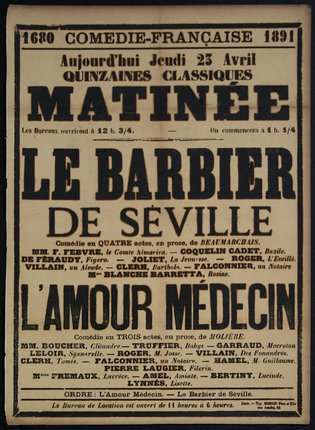This image features an old, off-white, slightly worn flyer entirely in French, adorned with black text of varying sizes. The flyer, bordered with a double black line, prominently showcases the years "1680" and "1891" at the very top along with the words "Comédie-Française." The largest text highlights "Matinée," followed by the titles "Le Barbier de Séville" and "L'Amour Médecin." The text details appear cluttered with names and roles, where the names of the actual people are bolded and their respective characters are italicized, suggesting this is an advertisement for theatrical productions. The style of the flyer, reminiscent of early 1900s design, signifies its age, complemented by its muted, yellowed background akin to old newsprint.